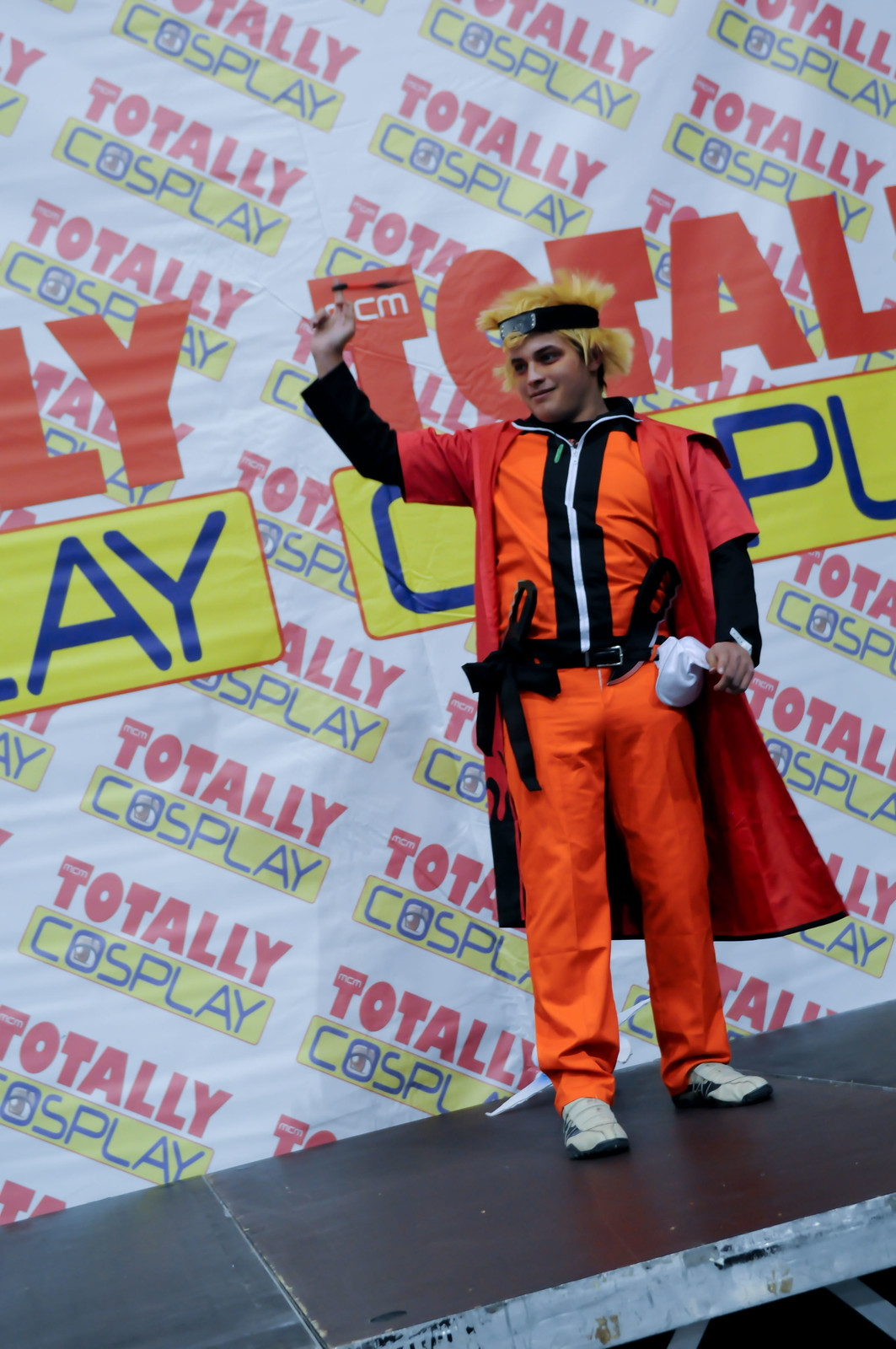A young man, dressed in an elaborate Naruto cosplay, stands confidently on a stage at a cosplay event. He sports a frizzy blonde wig with a black headband, reminiscent of the anime character Naruto. His outfit consists of an orange suit with a white zipper, orange pants, and a red short-sleeve overcoat adorned with black flames at the bottom. He raises his right fist in the air, triumphant, while his belt features what appear to be fake weapons. On his feet are white sneakers, completing his detailed costume. Behind him, a white curtain bears the event's name, "Totally Cosplay," repeated in red and blue text. The backdrop and the young man's smile create an engaging scene capturing the excitement of the cosplay event.